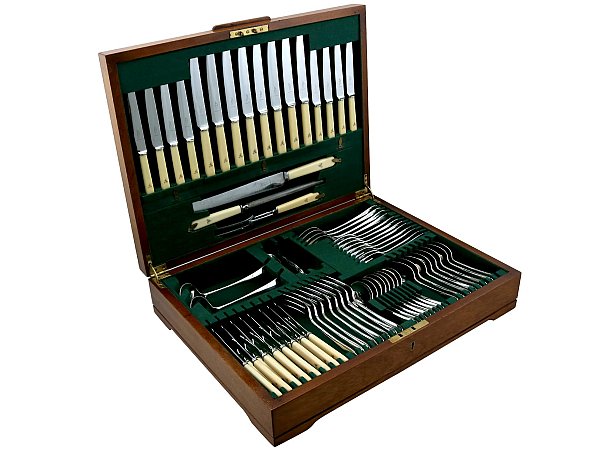This is a detailed product photograph featuring a comprehensive set of silverware housed in a dark, cherry wood briefcase-style box with a green velvet interior. The box is open, revealing meticulously organized utensils against a pristine white background. In the lid, various lengths of knives, including butter knives and steak knives, are securely tucked into designated sections. The bottom compartment of the box displays a collection of forks, spoons, ladles, and dessert spoons, all neatly arranged in their respective spaces. Additionally, the top left corner of the bottom section features serving spoons and forks. This image highlights the extensive and organized nature of the silverware set, making it ideal for product listings.